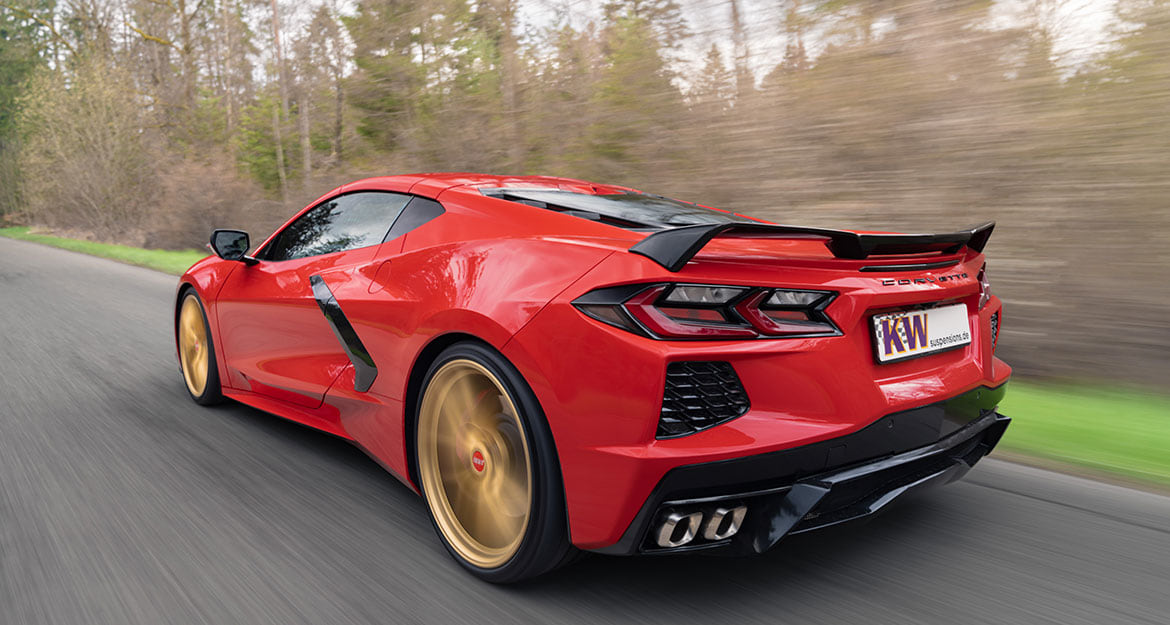The image features a red sports car, likely a Corvette, speeding down a black road. The car is distinctly in motion, as evidenced by the blur of its black tires with gold spokes and the surrounding scenery. Both the trees, which have mostly lost their leaves, and the grass beside the road appear blurry, emphasizing the car's speed. The car is detailed with black trim, including a black spoiler, lower bumper, air fin, and grille at the back. Notably, the vehicle has two exhaust pipes on the lower left side. The rear plate displays a white panel with a chequered flag in the top left corner and the letters "KW" in purple text surrounded by a yellow border. Additionally, there is some less distinct text on the right side of the panel, including "suspensions.de," and "Corvette" is written in black at the back. The windows are tinted dark, adding to the sporty, sleek look of the car.